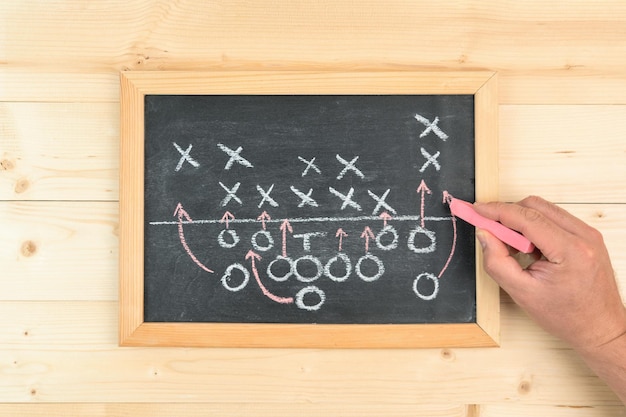This is a horizontally aligned rectangular image of a small chalkboard, centrally placed atop a light, unfinished wooden picnic table with four visible horizontal slats, some featuring darker brown knots. The chalkboard itself has a light wood frame, showcasing an array of white X's and O's, likely depicting a sports play, with pink and red arrows indicating movements, primarily directing the O's upwards. The lower section is divided from the top by a white line. Emerging from the lower right corner, a person's hand, presumably Caucasian, grips a piece of pink chalk, drawing an arrow connecting an O to an X. The casual, instructive scene suggests an informal strategizing moment or playful doodle reminiscent of planning a football play.